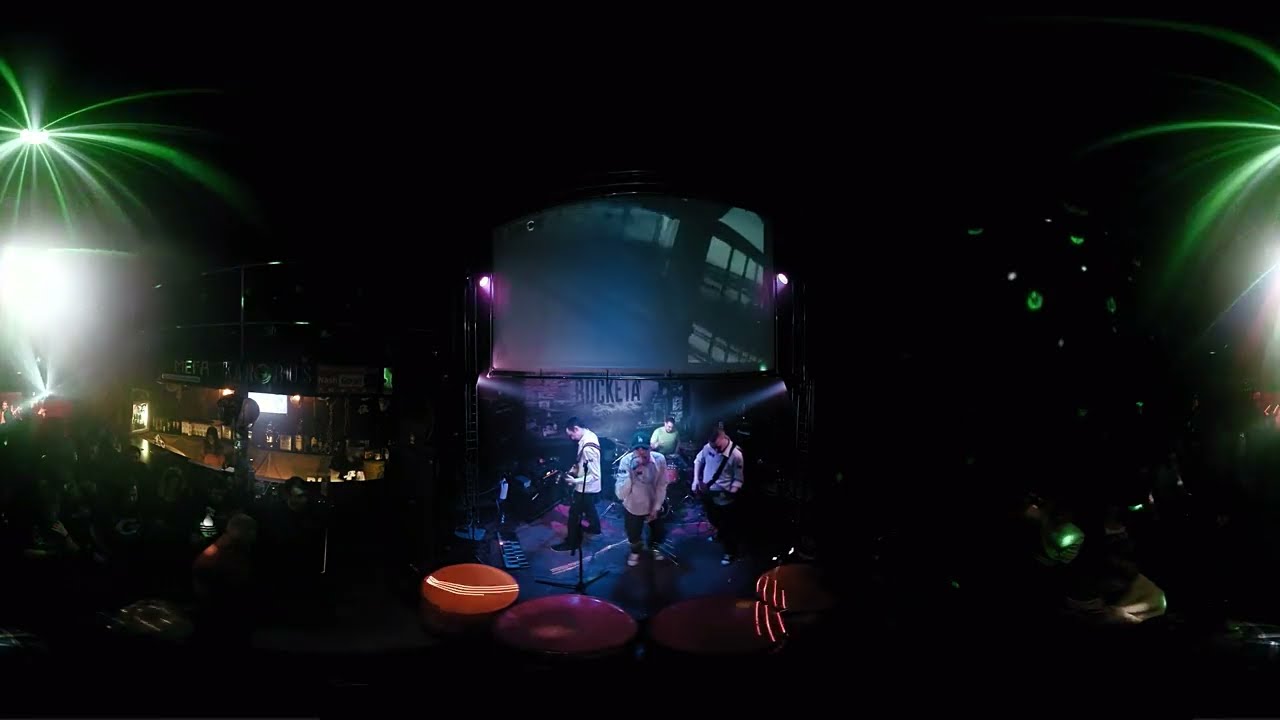This image captures a dynamic live band performance, showcasing four members on stage within a dimly lit venue, possibly a nightclub or a small concert hall. The focal point is the frontman, distinguished by a black hat, energetically singing into a microphone. Flanking him are two guitarists, both in white shirts with black pants. At the back, a drummer in a green shirt keeps the rhythm. The stage is faintly lit by unique lighting effects, including greenish palm-like illuminations and a red dot on the stage, possibly indicating the singer’s spot. On the right and left edges of the image, darkness envelops the scene, save for sporadic bursts of light and a spotlight on the right. The background reveals a bar area with visible bottles and two bartenders serving drinks. The word "Rakata" is displayed on the wall behind the band. The audience is partially visible, mingling in the darkened room.